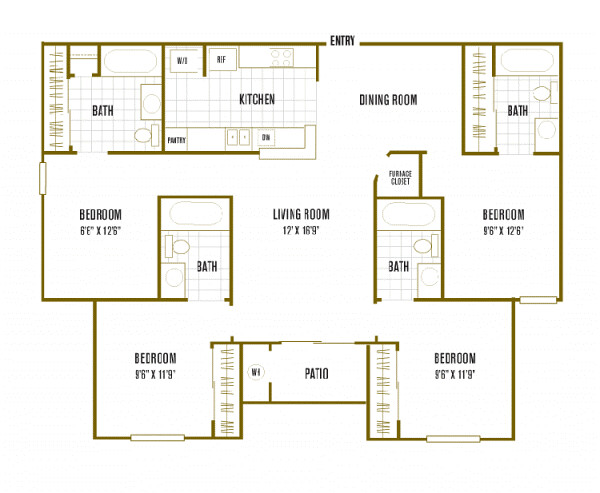This blueprint depicts a detailed layout of a residential dwelling. 

**Entry and Dining Room:** 
At the top of the blueprint, a long wall features a break labeled "entry," indicating the entry point into the dwelling. Upon entering, a resident would step into an open-floor plan dining room. This dining room serves as a hub, opening into a living room, a bedroom, and to the right, a kitchen.

**Kitchen Area:**
The kitchen, adjacent to the dining room, appears to have a sketched tile floor. Directly to the right upon entry is a cooktop or range, a refrigerator, and a partial wall. The partial wall has some unclear markings featuring a "W." Across from the cooktop, there's a pantry, which could be shelving, a cabinet, or a closet. To the left upon entry, there's a dishwasher (labeled "DW"), a counter, and a double sink.

**Living Room:**
From the dining room, walking straight through leads to the living room. This substantial rectangular space measures 12 feet by 16 feet 9 inches. Positioned between the living room and the dining room is a furnace closet, which features an angled edge door.

**First Bedroom and Adjacent Bathroom:**
Leading from the living room to the left (or right when entering the house), a small hallway leads to a bedroom measuring approximately 6 feet 8 inches by 12 feet 6 inches. This bedroom has a single window on the left side wall. Facing the front of the house from this room, there's an entry to a bathroom with a tile floor. The bathroom includes two closet doors on the left with clothing rods, a cabinet or shelf, a bathtub, a vanity sink, and a toilet positioned in the bottom right corner upon entry.

**Second Bedroom and Bathroom:**
Going back through the living room to the dining room and then accessing another bedroom directly across, it measures 9 feet 6 inches by 12 feet 8 inches. Positioned towards the back of the house, this bedroom features one window in the far corner (bottom right on the blueprint). Adjacent to it, there’s another bathroom with tile flooring, a single sink, a toilet, a bathtub, and closets with clothing rods.

**Additional Bedrooms and Bathrooms:**
There are two more bedrooms on either side of the living room, each measuring about 9 feet 6 inches by 11 feet 9 inches. The bedrooms have adjacent bathrooms featuring sinks, toilets, and bathtubs. They also each include closets with sliding doors and clothing rods, plus a single window centered on the wall facing the back of the house.

**Patio:**
Leading off the living room at the bottom of the blueprint are sliding doors opening to a "patio." The patio seems enclosed, though it is unclear if it is a screened room, deck, or balcony. There is also a label or icon next to it that is illegible at this resolution but may indicate additional features.

This blueprint offers a meticulous view of the residence, highlighting the interplay of its various spaces and functional areas.